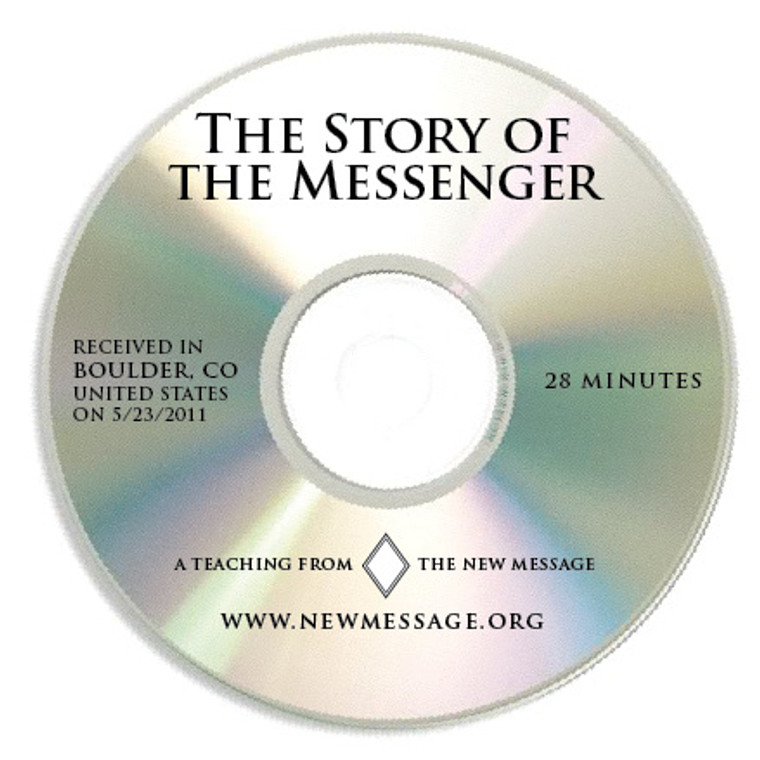The image depicts a metallic-colored CD floating against a stark white background, creating the impression of the disc suspended in a white void. The CD features an inner circle made of clear plastic acrylic. Black text is printed across the CD's surface: at the top, it reads "The Story of the Messenger." On the left side, the text states "Received in Boulder, Colorado, United States on 5-23-2011," while the right side notes "28 minutes." At the bottom, the text reads "A teaching from The New Message" followed by "www.newmessage.org" twice. The CD displays a spectrum of light, showing faint blurry hues of purple, blue, yellow, green, and pink. There is a single white diamond symbol at the bottom of the CD. There's no additional religious symbology or further explanation regarding the messenger or the content of the teaching.